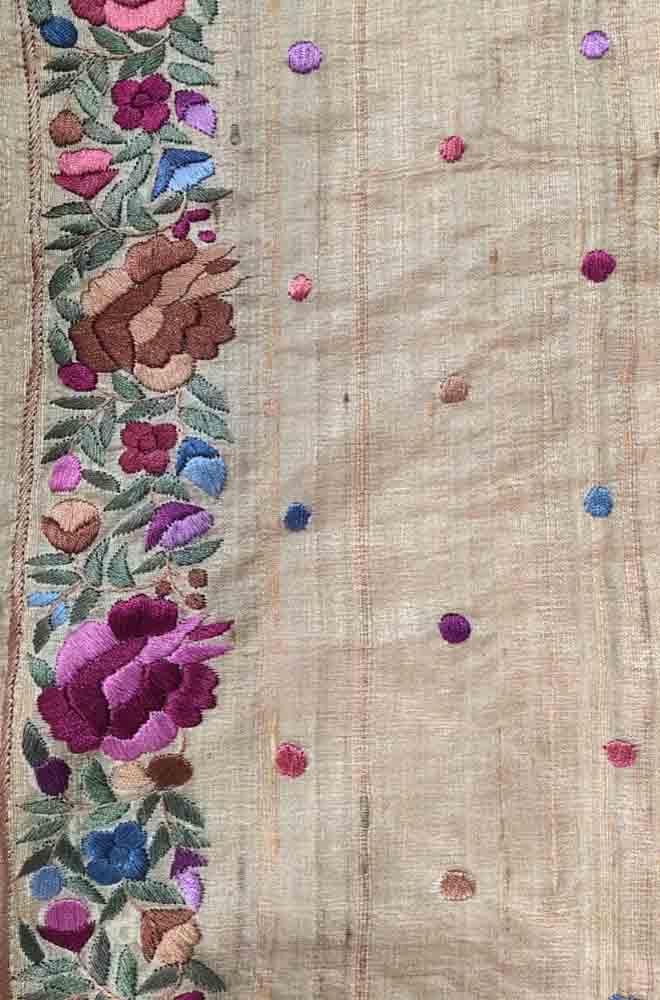This image features a piece of fabric, possibly an antique handkerchief, made with intricate detail. The background is a subtle gray or light beige, creating an understated canvas for the elaborate patterns that adorn it. The left side of the fabric showcases a narrow, vibrant border of multicolored flowers and leaves. Among these, large roses in shades of brown, tan, magenta, and pink stand out, interspersed with smaller flowers in purple, pink, and blue hues. Green leaves enhance the floral motif, creating a visually striking pattern. On the right side, a series of vertical brown streaks interspersed with evenly spaced, colorful dots—purple, pink, and blue—add a contrasting yet harmonious element to the design. The fabric's artistry and detailed sewing suggest it is handmade and lends it an antique, homemade charm.